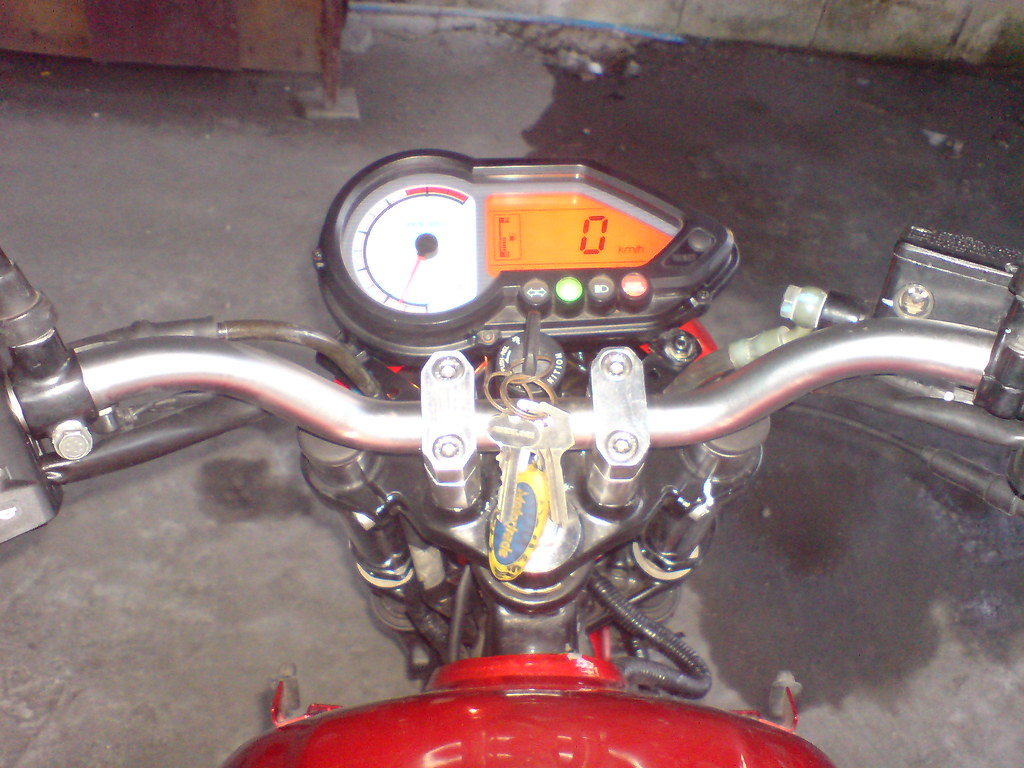The image depicts a basic two-wheeled vehicle, which could either be a motorcycle or a ride-on mower, making it challenging to identify. The handlebars are made of solid metal and lack visible grips. Prominent features include a gear shift indicator and a speedometer displaying both kilometers per hour and miles per hour, currently reading zero. Dangling from the vehicle are keys, next to a black ignition button. Below the speedometer are several buttons: one black, one red, one green, and another black.

Attached to the handlebars are two metal boxes, one on each side. A clamp and tubing extend from the front part of the vehicle to a red, shiny section, adding to the ambiguity regarding whether it is a motorcycle or part of a ride-on mower.

The vehicle is stored in what appears to be a flooded basement or garage, as evidenced by a large puddle of murky water spreading outward. The surrounding area is cluttered with a discarded blue item and an old piece of furniture. The wall in the background is heavily stained with moss and mold, suggesting prolonged exposure to damp conditions.